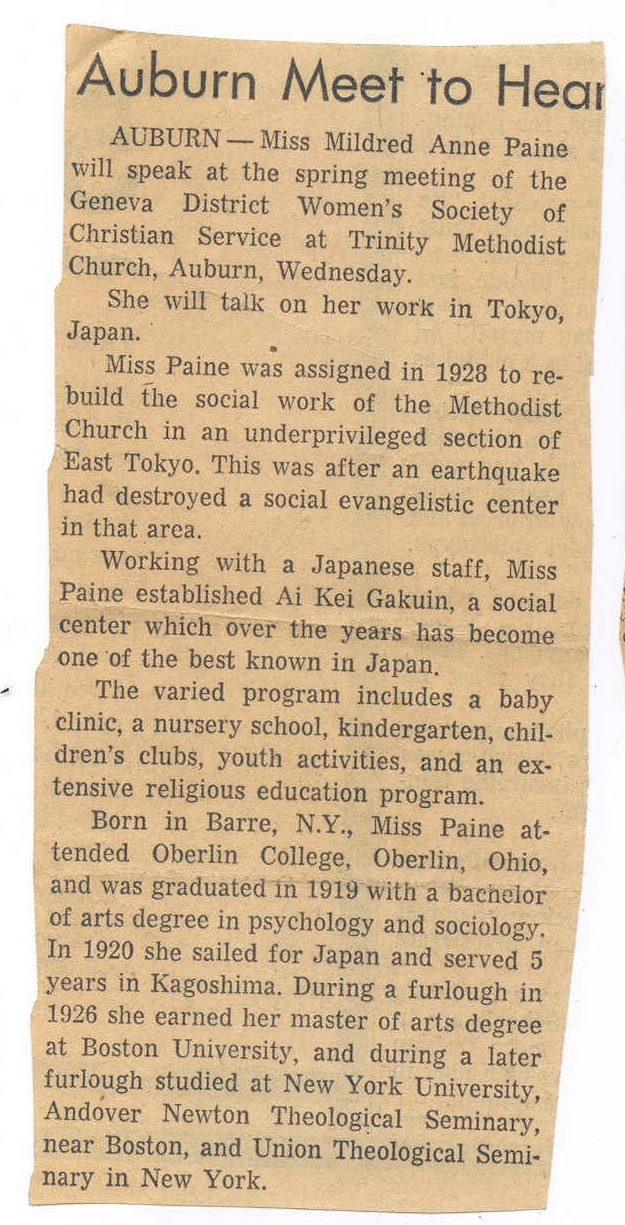The image is of an old, yellowing newspaper clipping, rectangular and densely filled with black text. The clipping, with jagged edges indicating it was cut from a larger piece, is titled "Auburn meet to hear". It highlights an upcoming event where Ms. Mildred Ann Payne will speak at the spring meeting of the Geneva District Women's Society of Christian Service at Trinity Methodist Church in Auburn, on Wednesday. The article details Ms. Payne's significant contributions to social work in Tokyo, Japan, where she was assigned in 1928 to aid in the rebuilding efforts for the Methodist Church in East Tokyo's underprivileged area following an earthquake that destroyed a social evangelistic center. Collaborating with a Japanese staff, she established IK Gakuin, a renowned social center offering programs such as a baby clinic, nursery school, kindergarten, children's clubs, youth activities, and extensive religious education. Born in Barr, New York, Ms. Payne graduated from Oberlin College in Ohio in 1919 with a Bachelor of Arts degree in psychology and sociology, and in 1920, she began her service in Japan, initially spending five years in Kagoshima. During a furlough in 1926, she earned a Master of Arts degree at Boston University, and during subsequent furloughs, she furthered her studies at New York University, Andover Newton Theological Seminary near Boston, and Union Theological Seminary in New York.